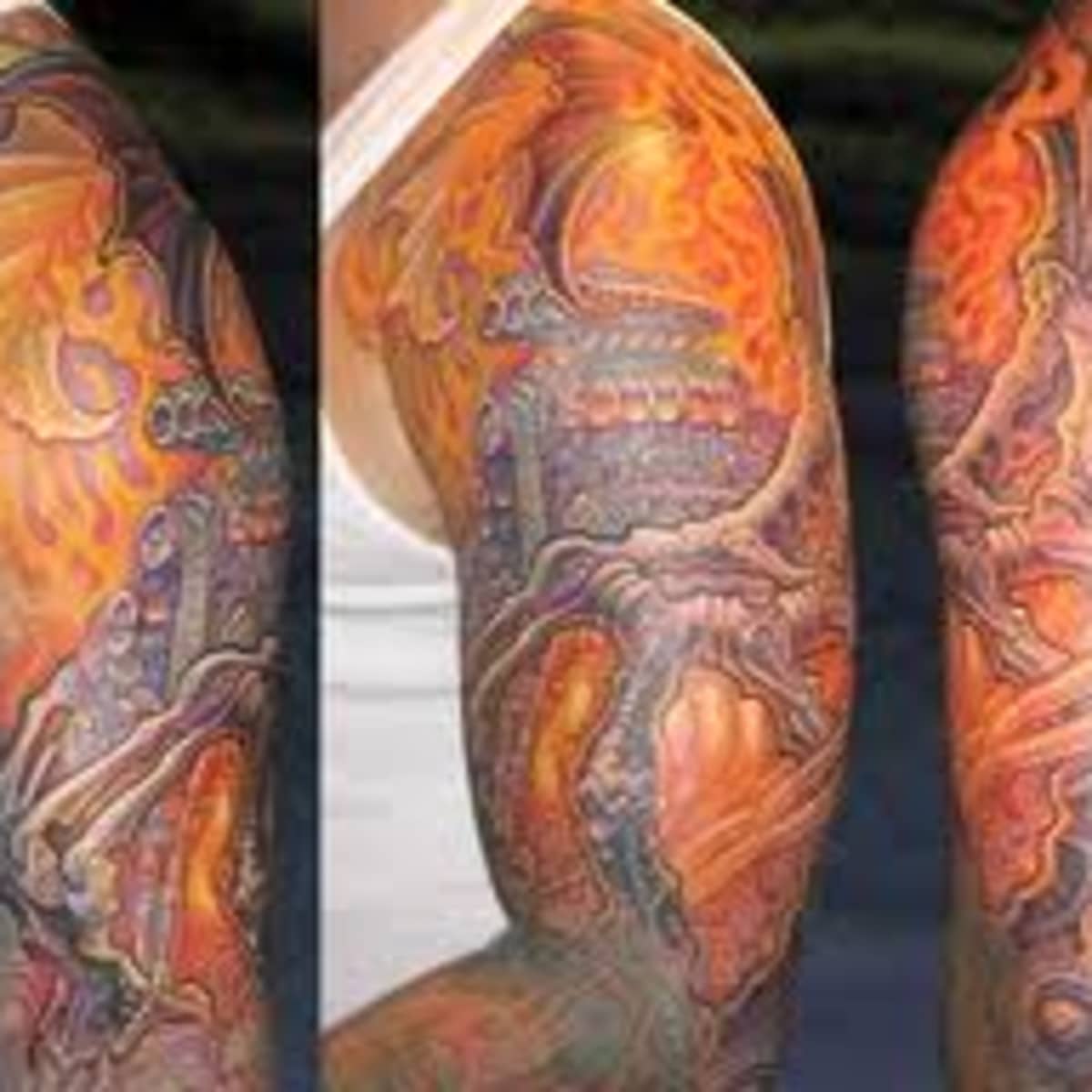The image features a man's heavily tattooed left arm, wearing a white tank top against a dark backdrop. The tattoos are detailed and intricate, covering the arm from the shoulder down to just past the elbow, with colors including black, white, gray, orange, red, yellow, blue, green, purple, brown, and tan. The presentation of the arm is broken into three sections: the left side shows the arm at one angle, while the middle and right sections are parts of a single continuous image, showing the arm from different angles. The tattoos incorporate complex patterns and lines, with some areas depicting flames in bright colors. The overall arrangement highlights different parts of the tattoo sleeve, showcasing the artwork from various perspectives.